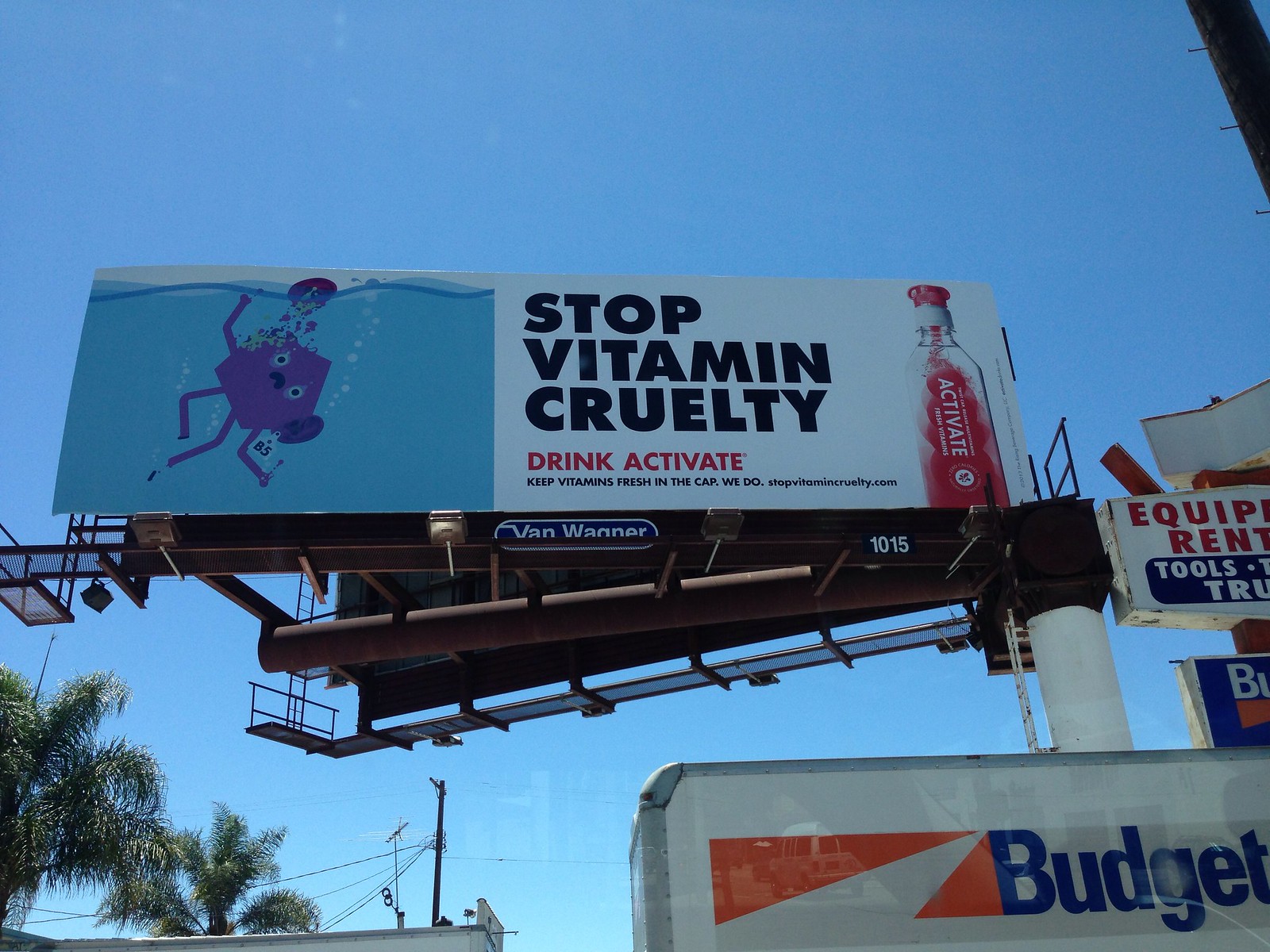The image features a slightly rectangular, horizontally oriented frame, capturing an upward perspective towards a vast, light blue, cloudless sky. In the bottom right corner, there is the roof of a moving truck, which is predominantly white with the word "Budget" emblazoned in blue on its side. Rising from behind the truck is a tall pole that supports two large beams extending horizontally to the left, which hold up billboards. The billboard facing the viewer is divided into two sections: the left side showcases a light blue background resembling water, featuring a small, purple, octagonal creature floating among bubbles. On the right side of the billboard, against a white backdrop, bold text reads, "Stop Vitamin Cruelty Drink Activate," with a vertically positioned bottle of Activate placed at the far right.